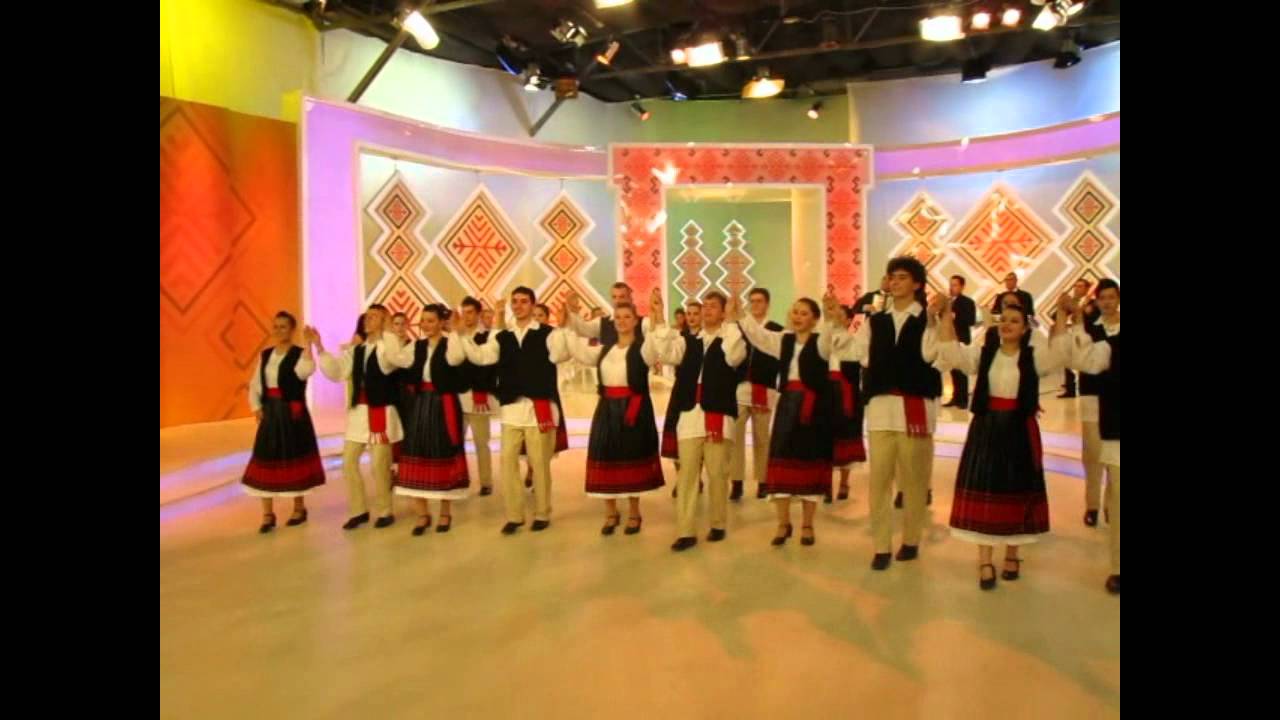A vibrant color photograph captures a lively scene within a studio, featuring a diverse group of traditional dancers, equally composed of men and women arranged in three or four rows. All dancers, numbering around a dozen, wear coordinated outfits: the women don white shirts with black vests and long black skirts adorned with red accents, paired with black pumps, while the men sport white shirts, black vests, beige pants with red sashes, and black shoes. They stand on a white floor, holding hands raised in the air, likely mid-performance. The background displays pastel-colored geometric patterns in hues of yellow, blue, purple, green, and orange, and the scene is illuminated by white studio lights from a dark ceiling. Musicians can be spotted playing instruments towards the back and to the right, enhancing the cultural ambiance of this exuberant dance event.